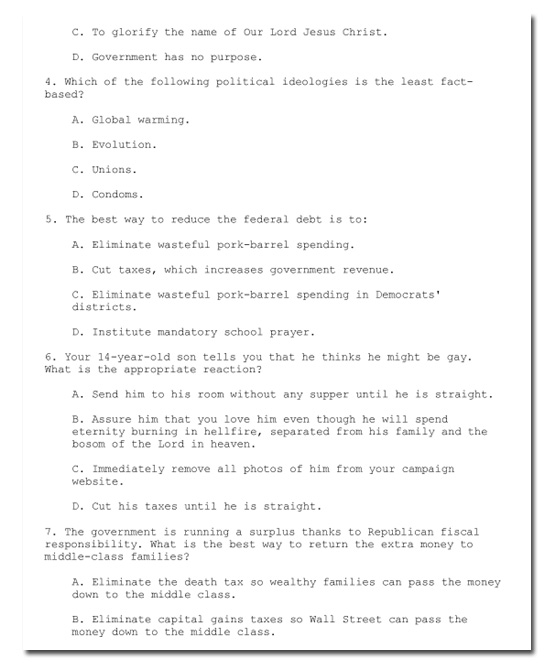The image depicts a highly organized document, likely a test or study material for a government or religion examination. At the top, the document begins with the heading "C. To glorify the name of the Lord Jesus Christ," indicating its religious context. This is followed by another section labeled "D. Government has no purpose."

The document further features a series of numbered questions, each accompanied by multiple-choice options. For example, question 4 reads, "Which of the following political ideologies is the least fact-based?" with options A (global warming), B (evolution), C (unions), and D (economics). Another listed question (question 5) is, "The best way to reduce the federal debt is to A, eliminate the wasteful pork barrel spending; B, cut tax, which increases government revenue; C, eliminate wasteful pork belly spending; or D, institute mandatory school prayer."

The text appears to be in a typewriter-style font, all in black, with standard spacing resembling MLA formatting. The questions are numbered and indented, giving the document a structured look. Additionally, the bottom-right edge of the paper seems to have a slight shadow, suggesting some thickness to the border.